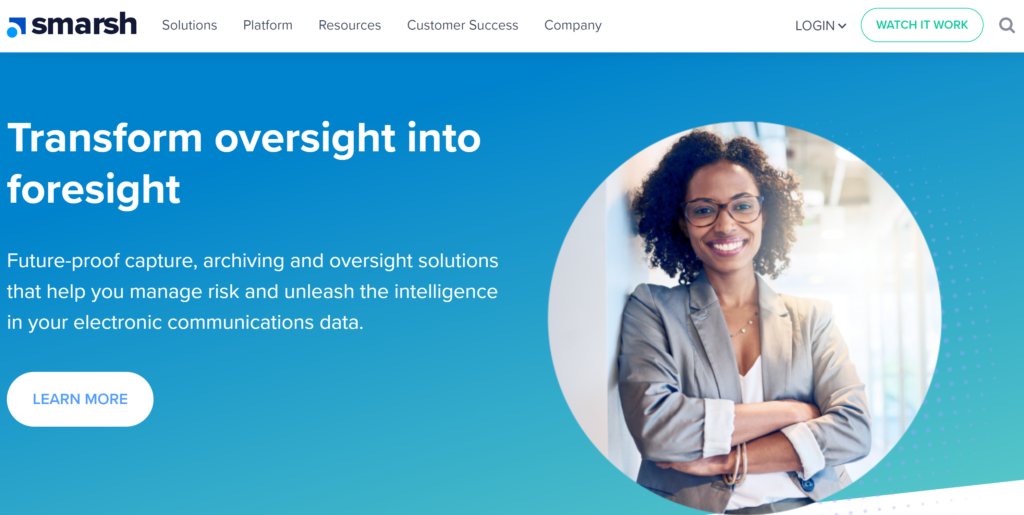The top left corner features the word "SMARSH" in black text accompanied by a logo consisting of a blue square. Inside the square, a white and blue circle is positioned near the bottom left. To the right of the logo, there are gray text labels that state: "Solutions," "Platform," "Resources," "Customer Success," and "Company." The top right corner includes a "Login" option and a button labeled "Watch It Work." Additionally, there's a gray magnifying glass icon.

Directly below, a blue banner displays the slogan "Transform Oversight into Foresight" in large, bold white text. Underneath the banner, a brief paragraph describes the services offered: "Future-proof capture, archiving, and oversight solutions that help you manage risk and unleash the intelligence in your electronic communications data." Adjacent to this paragraph is a white button with the text "LEARN MORE" in blue, all capital letters.

To the right of the text, a circular image showcases a woman with frizzy hair, wearing glasses, and smiling with her arms crossed. She is dressed in a gray suit, adorned with a necklace and bracelets.